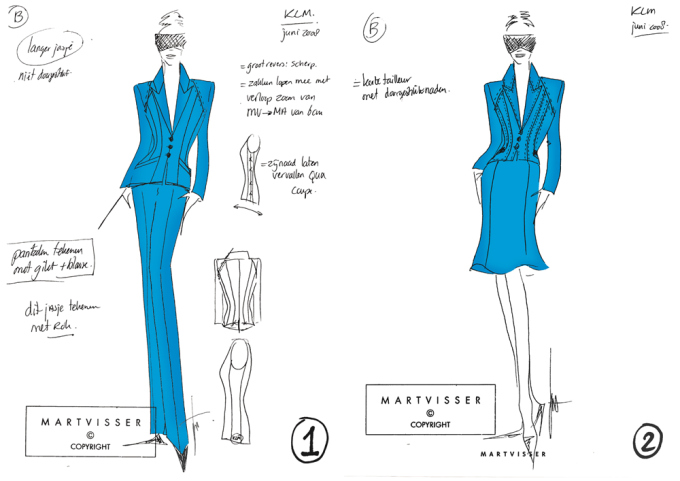The image showcases detailed fashion sketches likely created by a seamstress, dressmaker, or clothing designer. In the upper left corner, a handwritten letter "B" is circled with some illegible writing beneath it. Both sides of the image feature two almost identical drawings of a slender female figure. Each figure is wearing dark glasses and a power suit with distinctive blue jackets that have a low V-neck, square shoulders with shoulder pads, and a fitted waist accentuated by lines and three buttons down the front.

On the left side, the figure is dressed in matching blue dress pants and black shoes. The right side presents a version of the figure wearing a blue skirt, allowing her legs to show beneath. Both sketches have the word "Marta Visser" and a copyright symbol in the lower left corner and are numbered one and two respectively, indicating two variations of the fashion concept. These drawings are framed by handwritten notes, which might be in French, adding an authentic touch to the designer's creative process.